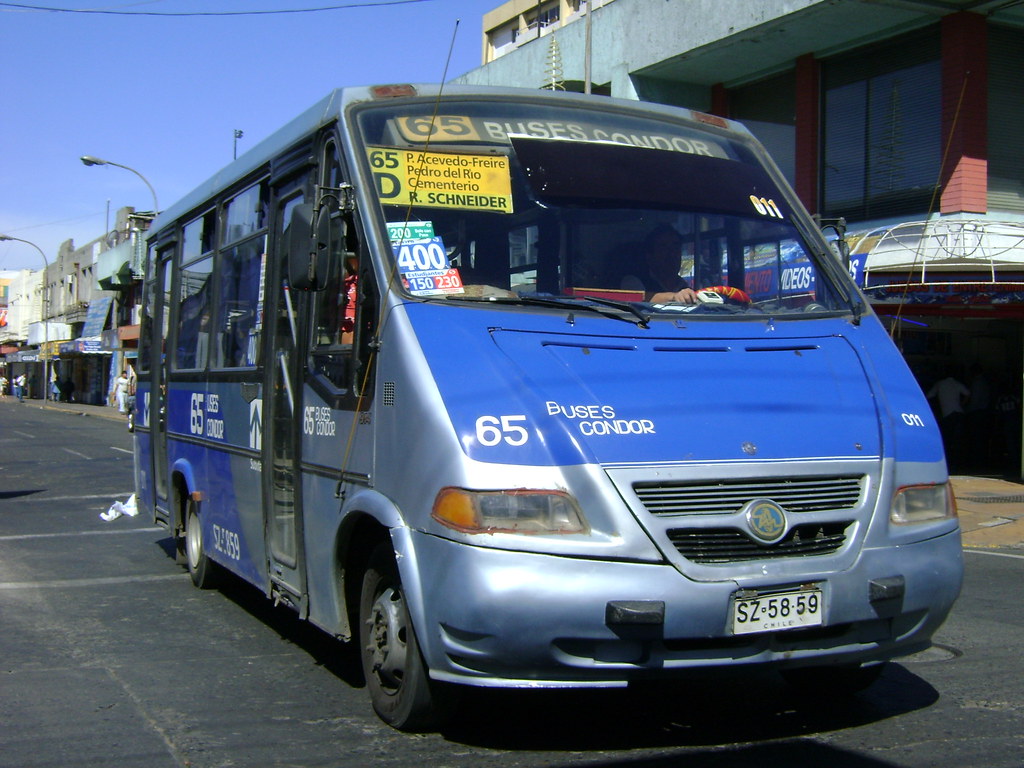This is a detailed color snapshot of a small metallic blue and silver van bus parked on a black asphalt street in what appears to be a suburban or small town commercial area. The front of the bus prominently displays the number 65 above the windshield and the words "Buses Condor." It features a yellow sign in the windshield marked "65D" and other text in Spanish, including "Pedro Del Rio" and "Schneider." The bus also displays its route number, 65, on the hood and the side. At the front, there is a white license plate with the number "SZ 58.59" in black text. Surrounding the bus is a line of one- and two-story buildings with white, gray, and light blue facades, indicating a bustling shopping area. The bus also has dark blue graphics and black trim. The weather is bright and sunny, casting clear shadows and highlighting the details of the scene, including some litter on the ground behind the bus.